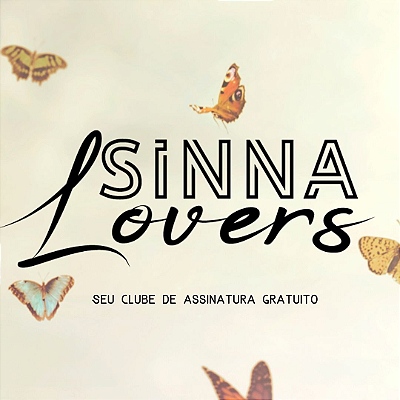This digital graphic features a background in creamish tan, adorned with colorful butterflies scattered across the design. The butterflies, totaling five, display a diverse palette: blue, yellow, orange, and green, creating a sense of liveliness and motion. Prominently centered in the middle of the image is the text "SINNAH LOVERS." The word "SINNAH" is presented in a standard typeface, while "LOVERS" is elegantly scripted in black cursive. Directly below, there is a subtitle in uppercase black letters, purported to be in Spanish, reading: "SUEL CLUB DE ASINATURA GRATUITO." The overall aesthetic suggests a simple yet visually engaging logo or promotional graphic.